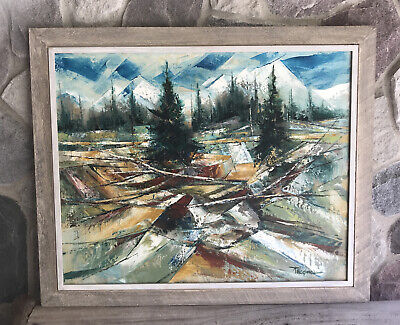The image features a piece of painted artwork hung on a gray stone wall. The artwork is encased in a brown wooden frame with a grayish inner border and a subtle white trim. The painting depicts a serene outdoor scene dominated by vibrant green pine trees and scattered broken branches. In the background, there are blue and white mountains suggesting a snow-capped range with pointy peaks. At the bottom right corner of the painting, there is a small black signature. The overall composition blends abstract and modern elements, adding to the intricate details and depth of the scene. Some white and brownish objects are also scattered throughout the landscape, though their exact nature is unclear. The contrast between the gray stone wall and the detailed artwork creates a striking visual effect.